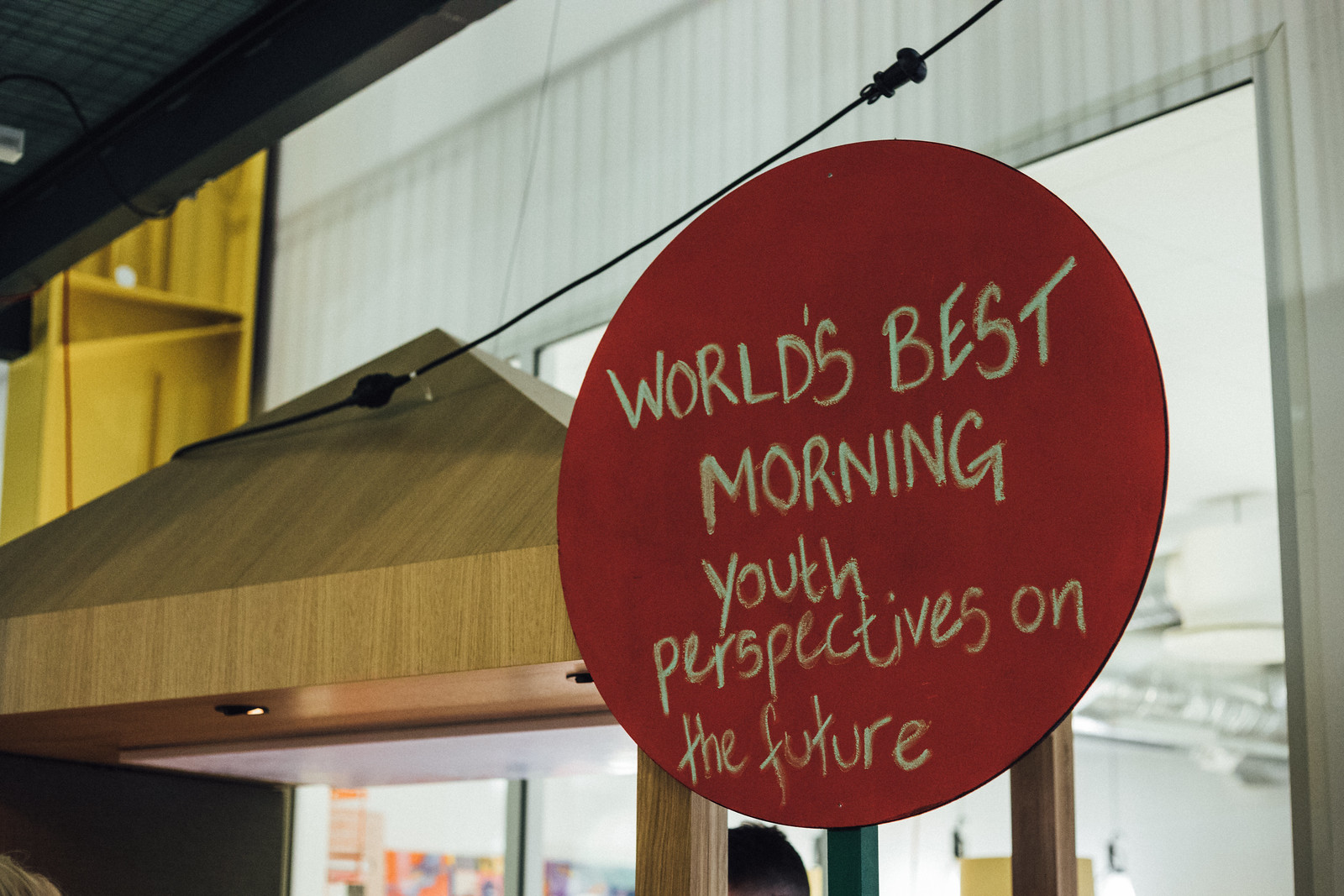The image depicts an indoor warehouse-like setting featuring a white corrugated wall and a black ceiling that may serve as a walkway for a second level. Dominating the foreground is a large, circular, red sign with white text that reads: "World's Best Morning Youth Perspectives on the Future." Attached to the booth, which has a wood grain and pyramid shape, is an electrical cable running towards the second-story level. Below the sign, partially obscured, is the back of a person’s head with dark hair. The booth appears to be supported by wooden boards and possibly includes small lights or switches underneath it. The scene is illuminated by natural light filtering through the windows, contributing to the overall brightness despite some areas’ industrial ambiance.